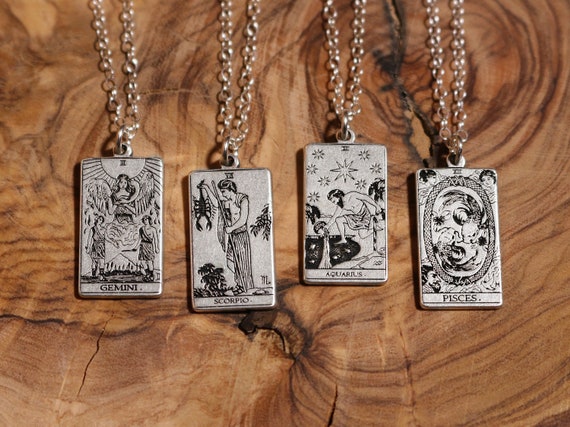The image showcases a set of four silver rectangular pendants, each representing a zodiac sign, elegantly displayed on a natural wooden surface with visible grain and knots. From left to right, the pendants are suspended from delicate silver chains with small links. 

The first pendant features "Gemini," depicting an angel with two figures in the background, likely symbolizing the duality of the sign. Next is "Scorpio," illustrated with a man holding up a scorpion by its tail. The third pendant, labeled "Aquarius," shows a bearded man pouring water, evoking the water-bearer imagery. The final pendant represents "Pisces," with a depiction of two fish, and includes human faces in each corner of the design.

The overall image is set against a light brown wooden surface with dark green tones, enhancing the natural aesthetic and highlighting the intricate silver and black line art details of each pendant.